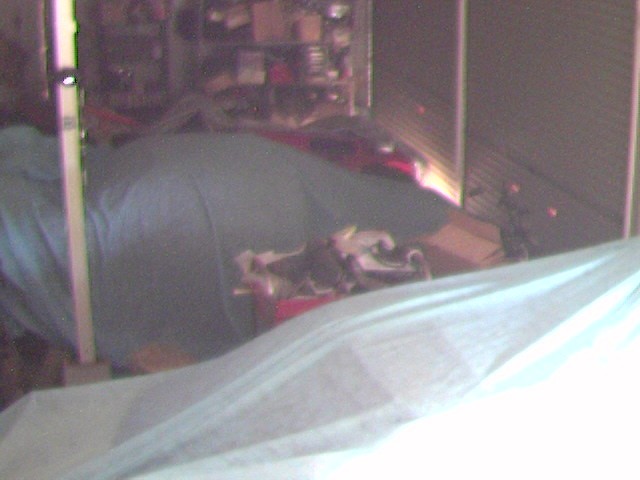This grainy, soft-focus photograph captures the interior of a cluttered storage garage. In the immediate foreground, a car is covered with a white cloth, its form barely discernible beneath the fabric. Positioned centrally in the room, another car hides beneath a darker cloth cover. A white pillar stands between the two shrouded vehicles. In the background, shuttered doors are drawn down, with a bright sliver of light streaming in from beneath one of them. The far wall features a cluttered shelf, crammed with boxes and indistinct items. In front of these shelves, a partially visible red machine—possibly another vehicle—emerges from the shadows, only partly uncovered. Additionally, a bicycle can be seen amid the disarray, along with more boxes stacked between the two covered cars, adding to the overall sense of organized chaos within the space.